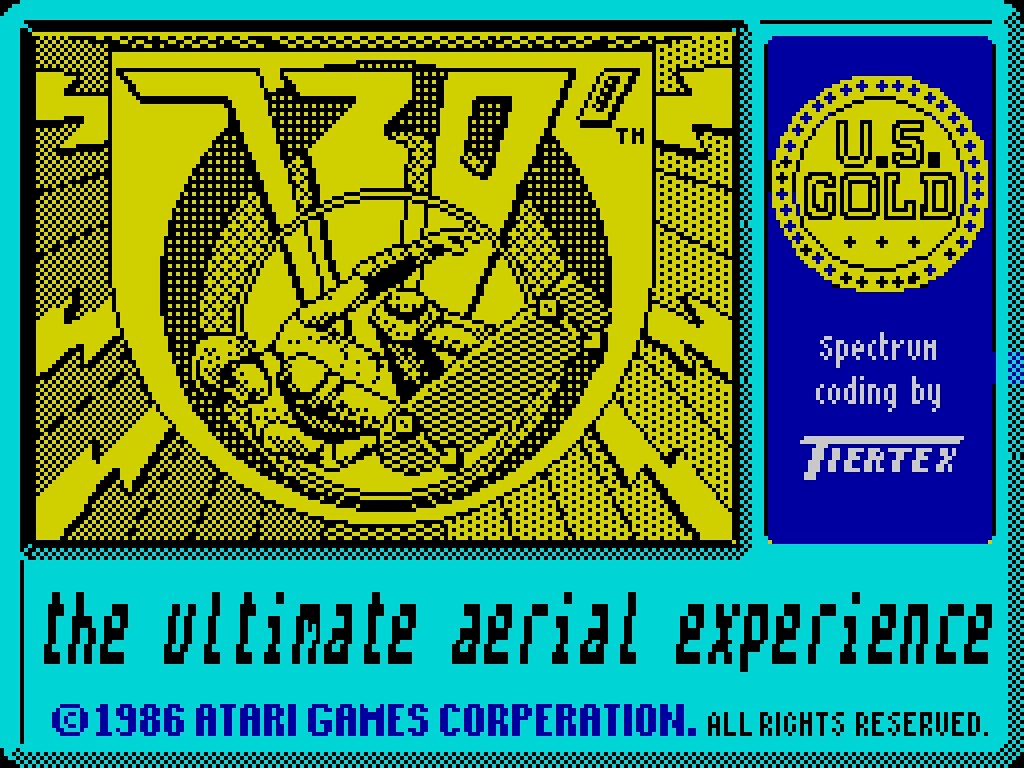The image is a vibrant graphic for a video game, prominently featuring a dynamic illustration of a skateboarder mid-trick. The background is a striking blue-turquoise color that sets a lively tone. Dominating the upper part of the image is a black and yellow digital design depicting a skateboarder with bent knees, his body leaning over his right leg. The skateboard is shown from beneath, with all four wheels visible. Above the skateboarder is the number "730°" followed by "TM". 

To the side, there is a gold emblem stating "U.S. Gold," set against a purple backdrop that also features the text "Spectrum Coding by Tiertex" in white letters.

At the bottom of the graphic, a bold slogan reads "The Ultimate Aerial Experience." Beneath this, in blue text, is a copyright statement: "© 1986 Atari Games Corporation". Below that, in black, it states "All Rights Reserved." 

The overall design is complemented by a dynamic lightning bolt pattern emanating from the skateboard, adding energy and movement to the illustration.